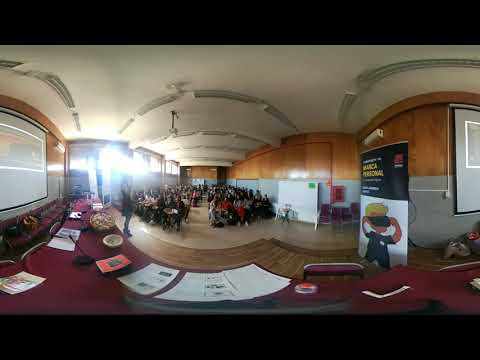The image captures the interior of a conference room, styled with both modern and classic elements. The ceiling is white with a mix of beige tones and lined with various, yet turned-off, fluorescent lights. The walls are adorned with light brown wood paneling on the top and painted a light gray on the bottom. In the foreground, a semi-circle table draped with a rich burgundy tablecloth is positioned, extending from left to right. The table is cluttered with a variety of white papers, charts, microphones, and a conspicuous poster featuring a blonde cartoon boy wearing a black eye mask. Mixed folding chairs with burgundy cushions sit at the table, facing towards the center of the room. The floor is covered in wood panels, complementing the warm tones of the space.

Several people are seated in rows, resembling a classroom or lecture hall setup, with a central aisle dividing the seating area. Light streams in from behind, possibly through windows, enhancing the natural warmth of the space. A stage, elevated by wooden steps, hosts a speaker—a lady addressing the attentive audience. The overall ambiance suggests a formal yet inviting environment, suitable for presentations, conferences, or lectures.